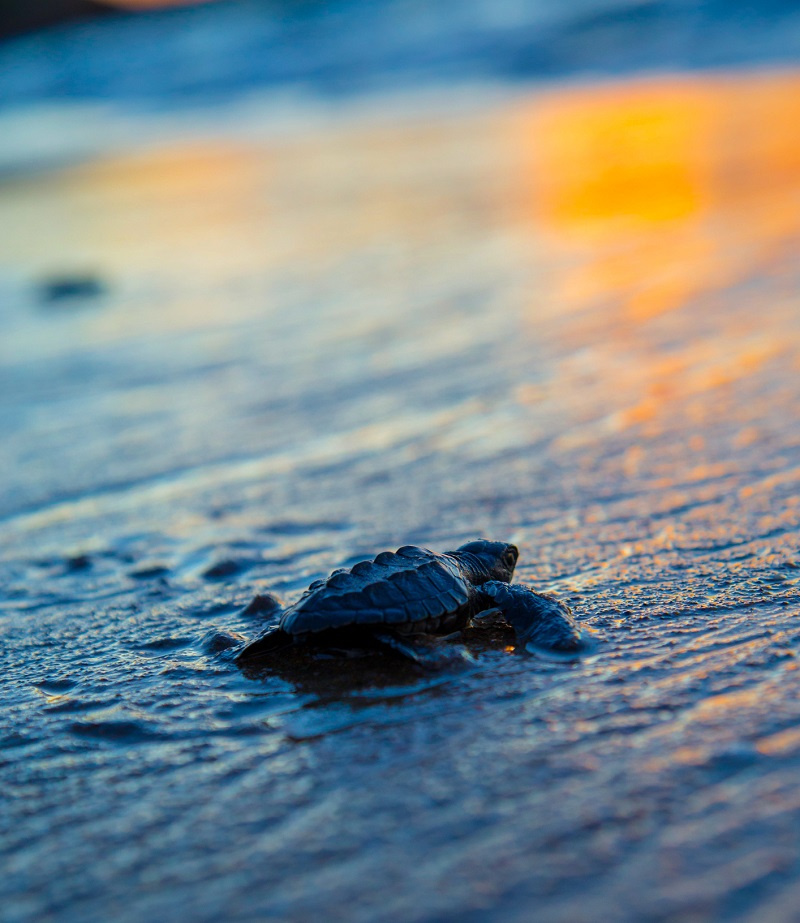The image captures a poignant scene of a solitary beached turtle on a seashore, surrounded by the soft hues of ocean blue, yellow, and lighter gray-blue. The turtle, which appears small yet indeterminate in size due to the lack of a comparison object, is facing right, with one of its big flippers extended in that direction. Its dark, unmarked shell glistens subtly under the hint of sunlight seen in the top right corner, casting a golden-yellow reflection on the wet, grayish-blue sand. The background remains artfully blurred, suggesting an early morning or sunset glow with hints of blue water and possibly orangey-red tones. The turtle seems to be struggling slightly on the wet, muddy sand, creating a striking focal point in this atmospheric and intimate capture.